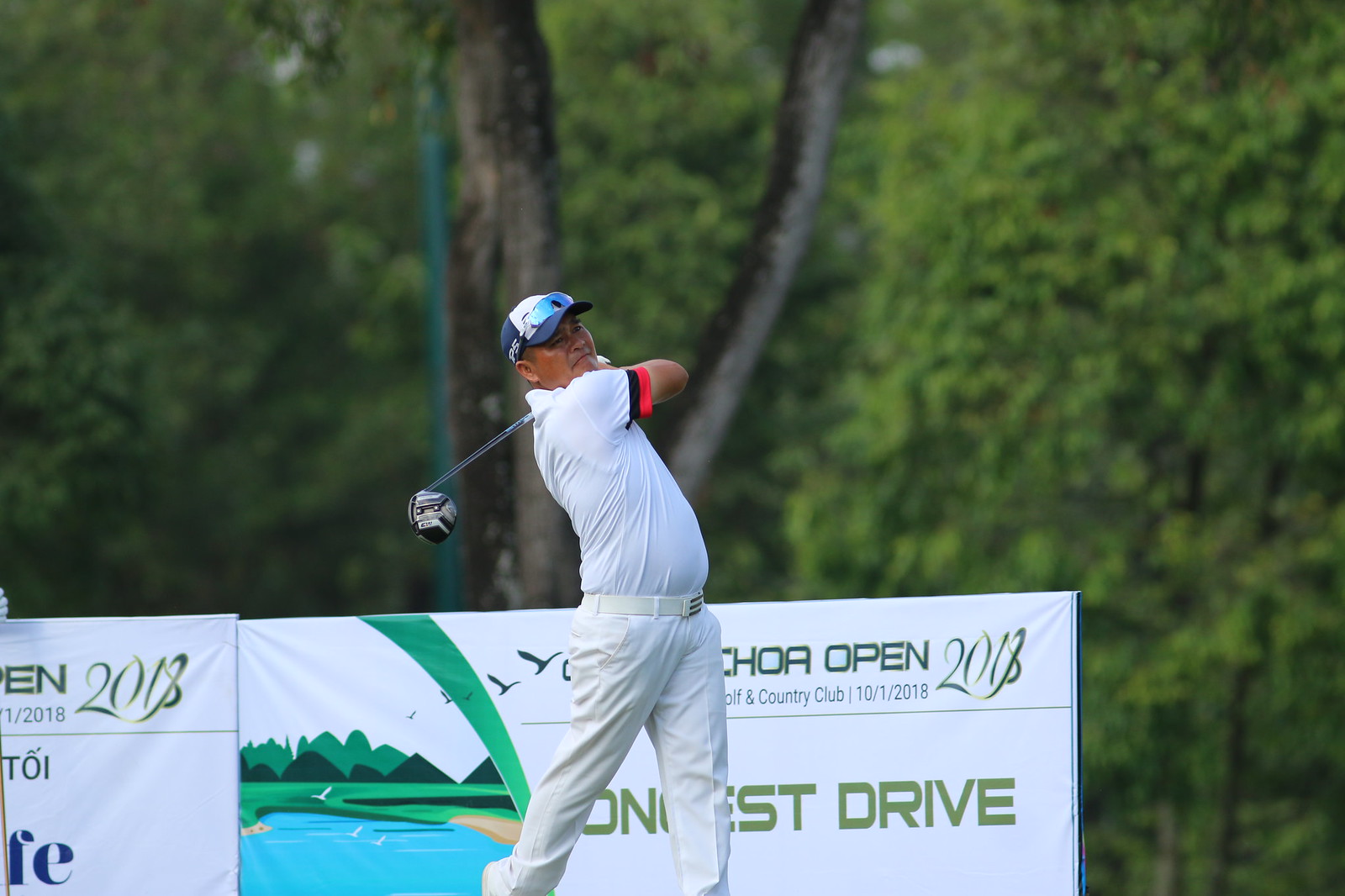In this vibrant outdoor scene captured during daylight, a golfer stands prominently in the center of the image, having just completed his swing. He is poised with his club resting behind his neck and is looking off to the right. The golfer is dressed in white pants, a matching belt, and a white short-sleeved shirt accentuated by red and black trim on the sleeve edges. He also sports a blue and white baseball cap with sunglasses perched on its bill, casting a shadow over his face. 

Behind him, various signs are partially visible, signifying an event that took place in 2018, including text indicating "CHOA Open 2018," referencing a golf and country club event that occurred on October 1, 2018, with a mention of "longest drive." The background is lush with greenery, featuring abundant foliage, trees, and tree trunks. Additionally, the scene includes a lamppost and a detailed artistic depiction of a golf course, complete with a pond and a sand trap, enhancing the immersive outdoor setting.